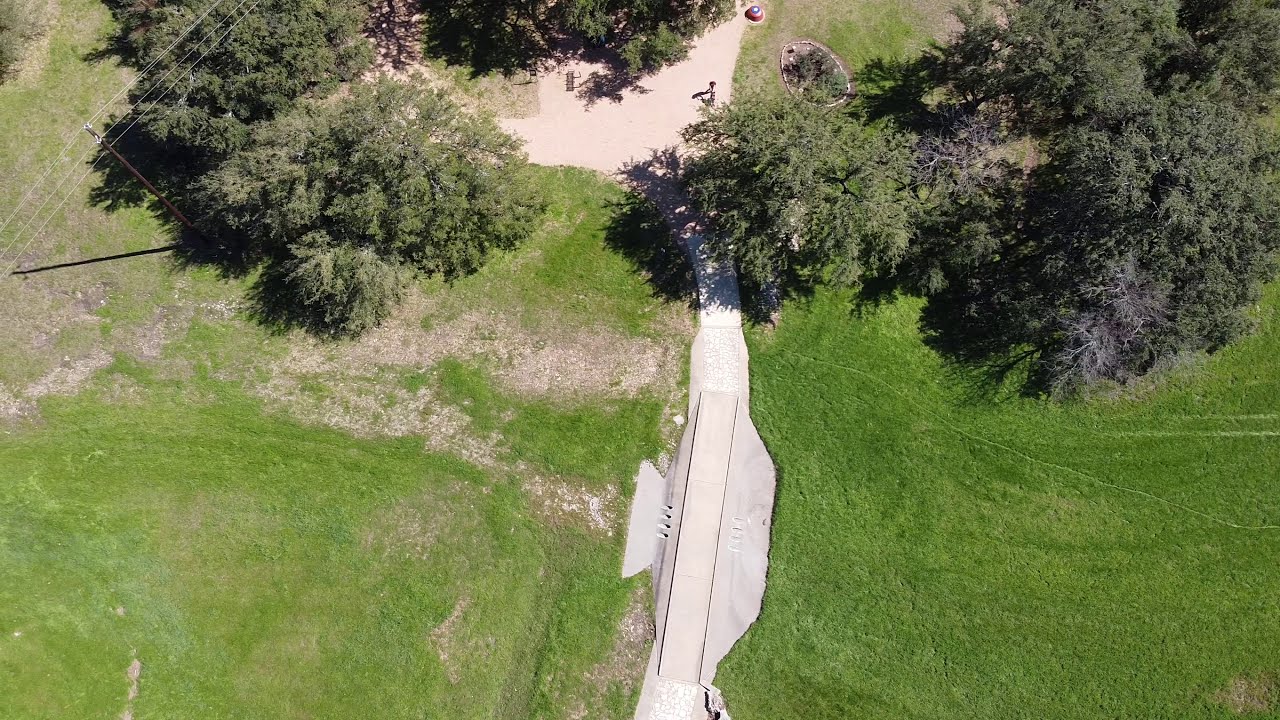This aerial photograph captures a detailed scene of a grayish stone or concrete path, potentially a bike trail or pedestrian walkway, meandering through an expansive grassy area. The path features cobblestone-like sections and leads to a central open space, possibly a gravel or dirt parking lot. To the left and right of the path, vibrant green grass is intermittently broken by patches of exposed dirt and rocks. Alongside the path, there is a small parking pullout or pullout section, a bridge with drainage culverts underneath it, and a distinct flower bed encircled by stones. The grassy area also contains a mix of live trees and scraggly dead trees, providing a diverse canopy. There are utility poles with power lines weaving diagonally across the scene. In the top segment of the image, a few human artifacts are visible, including a red circular object with a blue cap and white star-like shape, likely a waste receptacle, and a bench. This image encapsulates a harmonious blend of natural and man-made elements within the landscape.